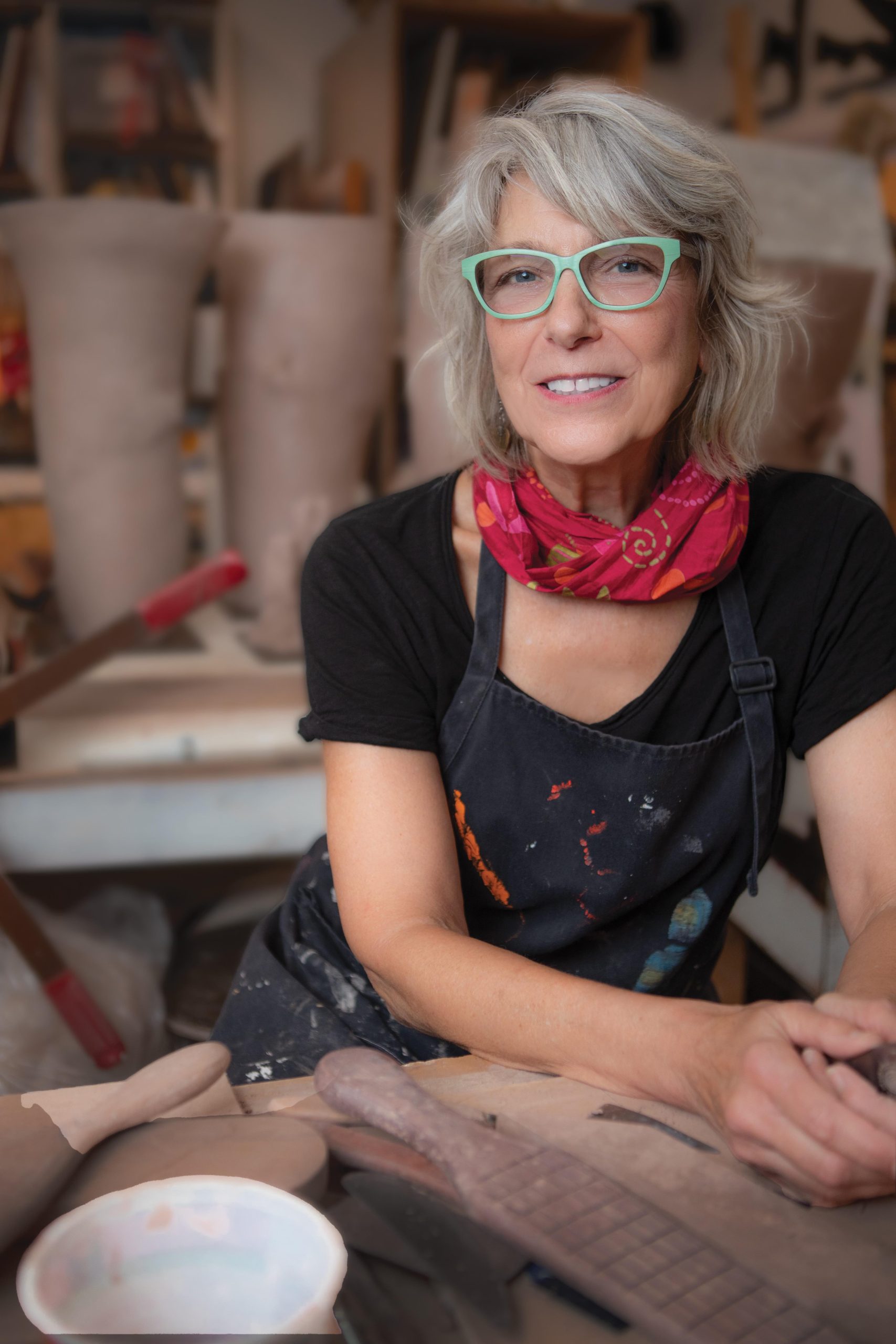In this vibrant studio photograph, a slightly tanned, white woman, exuding artistic flair, is captured mid-smile as she sits in front of a wooden workbench cluttered with various pottery tools and supplies. She is dressed in a paint-splotched dark blue or black apron over a short-sleeved black V-neck t-shirt, accompanied by a bright red scarf adorned with pink and orange designs wrapped around her neck. Her shoulder-length, shaggy gray hair frames her light teal, cat-eye glasses. Her hands are clasped together on the table, surrounded by tools likely used for working with clay, a white bowl possibly for keeping the clay moist, and a brush. In the background, other workbenches and urn-like clay objects add to the creative atmosphere, hinting at the bustling, artistic environment she thrives in.